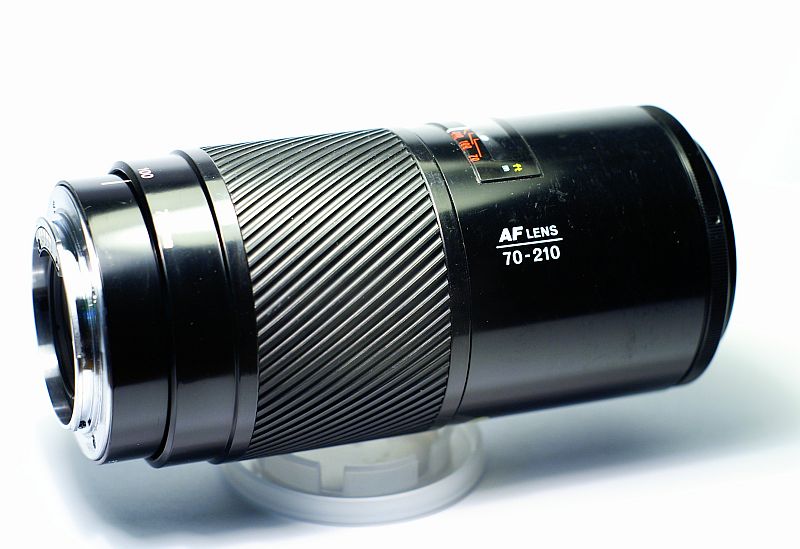This photograph depicts a close-up view of a black, cylindrical camera lens, reminiscent of those used by professional photographers, resting upright on a round, white circular base. Set against a brilliantly lit, plain white background that merges seamlessly with the table surface, the lens casts a distinct shadow. The lens features intricate details, including gray stripes along segments of its shiny black frame, which is designed with rotating and adjustable elements to modify the focal length and aperture. The front of the lens reveals the glass element, while along the side, there is white text reading "AF Lens 70-210," adding a touch of precision and specification to the image.